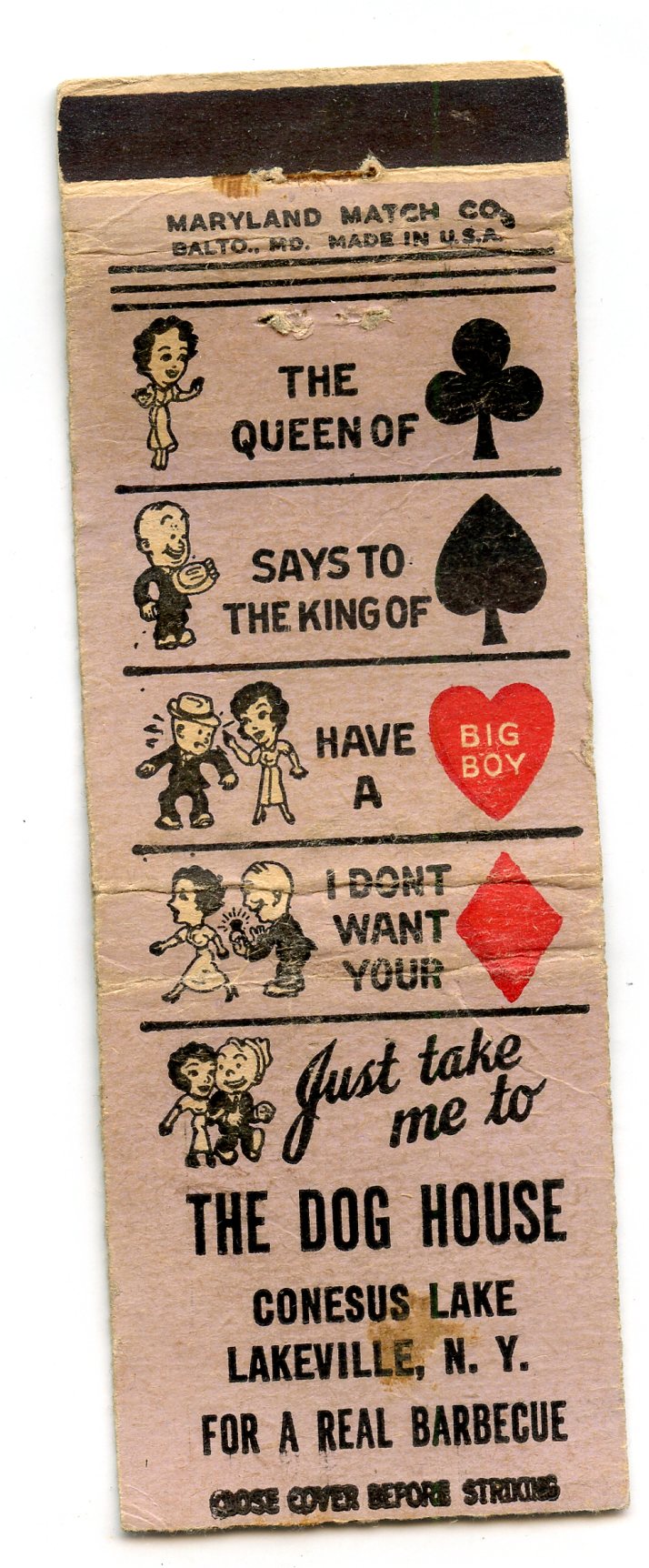This vintage matchbook cover, open vertically, advertises "The Dog House" restaurant at Canesius Lake, Lakeville, New York, known for its real barbecue. At the very top, it reads "Maryland Match Company, Balto, Maryland, Made in USA," potentially with a rusted staple. The cover features cartoon-like illustrations depicting a humorous dialogue between a husband and wife, divided into several sections by black lines. The first section has an image of a woman labeled "The Queen of Clubs," followed by a man labeled "The King of Spades" in the second section. The third section shows a heart with the words "Big Boy" inside. The fourth section, with the woman walking away, reads, "I don't want your diamond," highlighting her pointing to the man holding a diamond ring. The final section depicts them arm-in-arm with the caption, "Just take me to the Dog House." Poker card symbols for clubs, spades, hearts, and diamonds visually accompany the text. The matchbook also carries a safety warning: "Close Cover Before Striking."